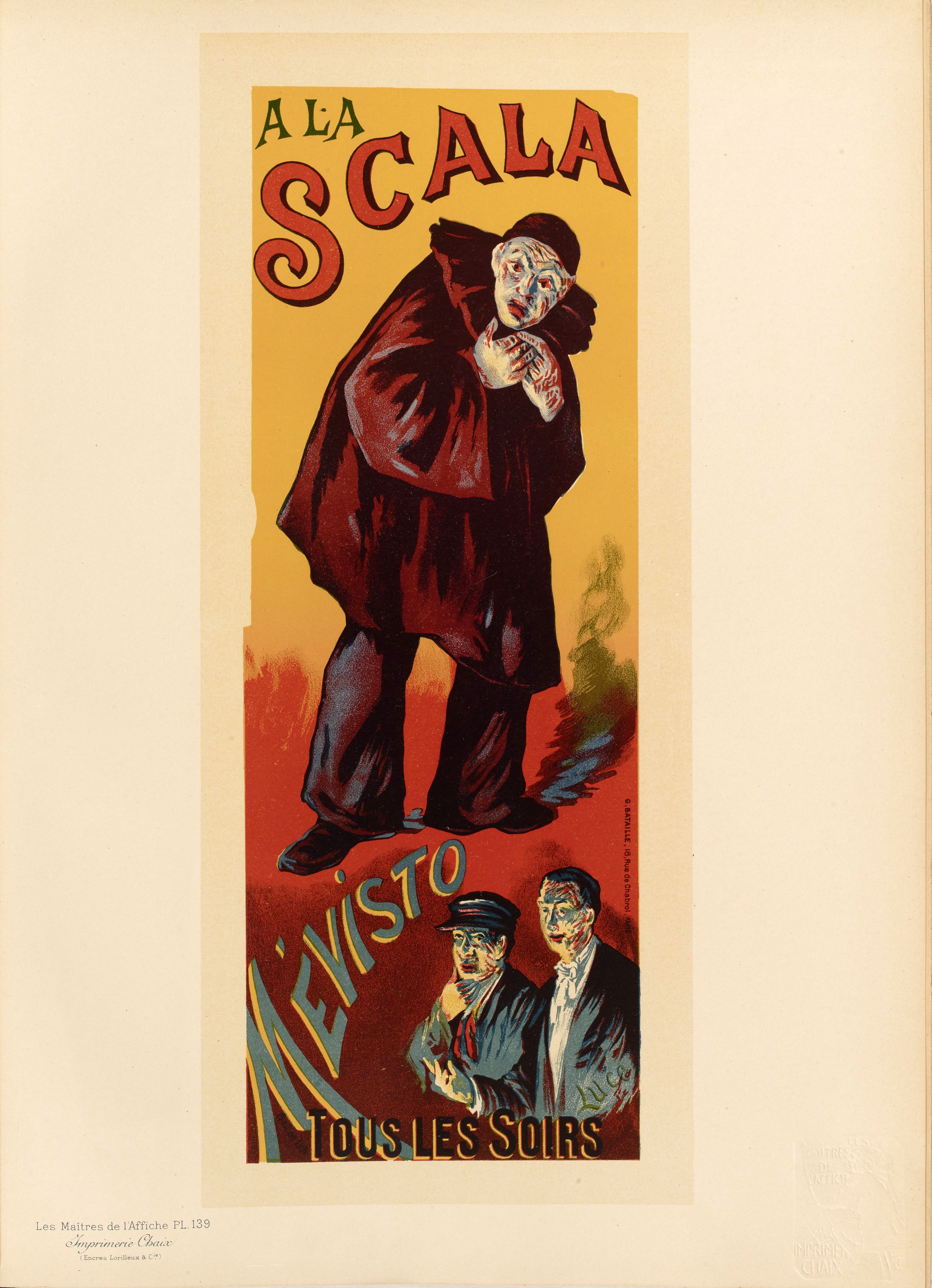The image appears to be a tall, vertically aligned poster with a vibrant pink background. Fine, unreadable black text is located in the lower left corner. Central to the composition is a colorful vertical rectangle set against a yellow background at the top, transitioning to red at the bottom. Dominating the upper portion of this inner rectangle is an eerie figure wearing a dark red top and reddish-black pants, reminiscent of a clown. The figure's face, resembling a mask with white, brown, and gray lines, contributes to its menacing aura. Above this figure's head, text reads "A-L-A" in green and then "S-C-A-L-A" in red. 

The lower half of the inner rectangle features two men whose upper torsos are visible, each sporting mask-like faces. The man on the left wears a black hat while the man on the right has short brown hair; both are clad in black jackets. The word "M-E-V-I-S-T-O" appears near these figures, arranged diagonally. Finally, an inscription at the very bottom of the poster reads "T-O-U-S L-E-S S-O-I-R-S." The overall effect and style suggest it is an artwork potentially intended for display in a museum or similar venue.